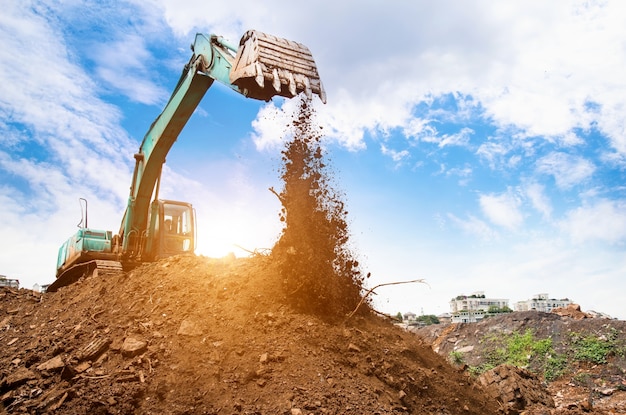In the foreground of the photograph, a well-worn green excavator with a silver-tipped arm is actively at work, its bucket tilted upside down to release dirt onto a substantial pile of soil filled with rocks, sticks, and debris. The arm, covered in chipped green paint, reveals the excavator’s age and wear. The scene captures the action as earth spills from the toothed bucket, adding to the mound beneath. The image is taken on a sunny day under a vibrant blue sky crowded with large, white clouds. To the right, gray windowed buildings stand on a predominantly dirt-covered hill, while possible ruins of stone buildings, barely discernible, are situated in the distant left background. Scattered grass patches can also be seen on the right side of the frame, adding a touch of greenery to the otherwise construction-dominated landscape.